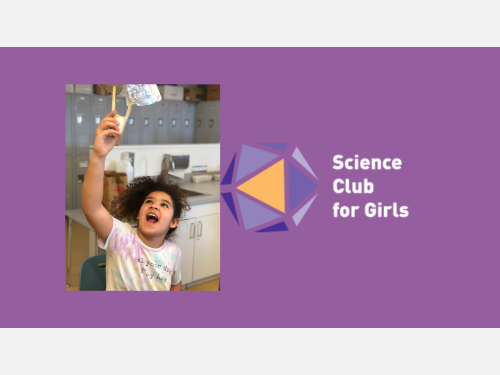The image features a bold and inviting sign for the "Science Club for Girls," emblazoned in crisp white letters on a vibrant purple background. The sign is accentuated by a dynamic geometric shape in shades of purple and orange to the left of the text. Adjacent to the shape, on the far left, is a lively photograph of a girl in a classroom laboratory setting. The girl is captured in a moment of genuine excitement, her face beaming as she holds a scientific device aloft with both hands, gazing at it with wonder. She is dressed in a light-colored tie-dye shirt which appears to have the words "Your Dog" printed on it, though the text is somewhat blurred. Her long, dark, and frizzy hair frames her face, adding to the charming and spirited atmosphere of the image. The background offers a glimpse of the classroom environment, with lockers faintly visible in the far distance and a counter with a sink, covered by a cloth, suggesting a typical, bustling school laboratory.